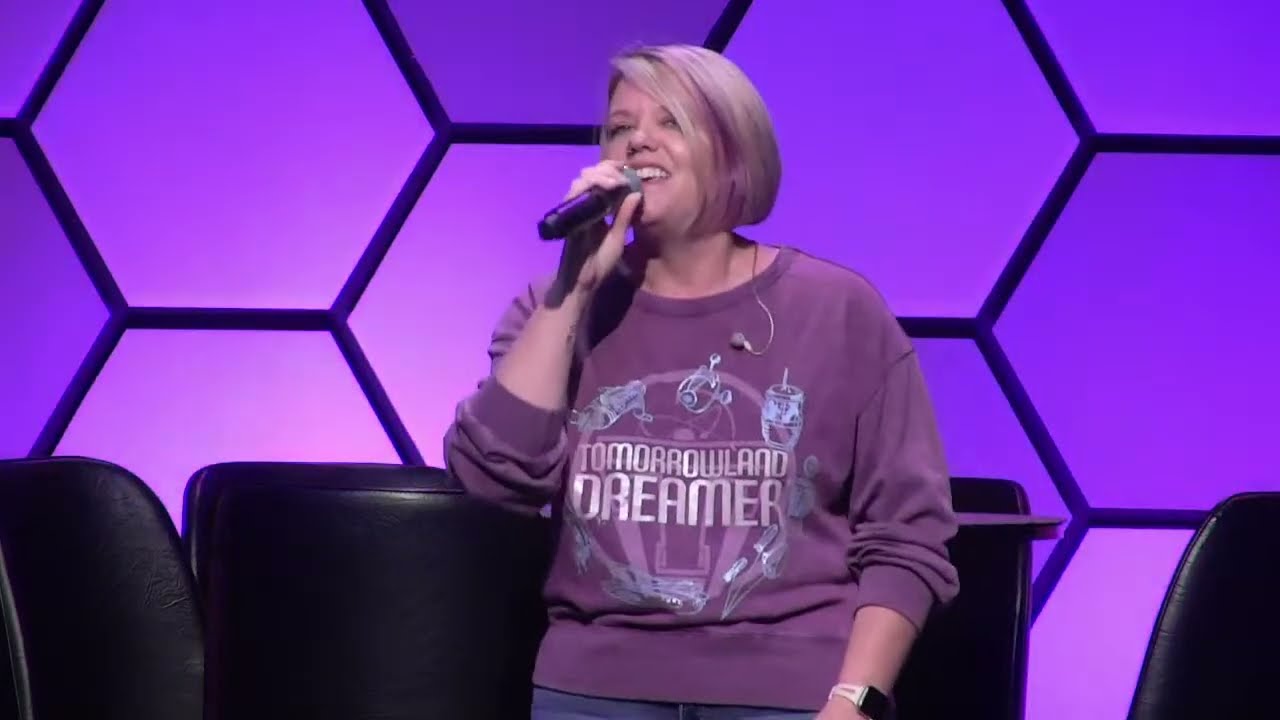The image captures a Caucasian woman, likely in her late 40s or early 50s, with a chubby face exuding a cheerful demeanor. She embodies a quintessential Midwestern mom appearance, sporting chin-length blonde hair with a striking purple streak down the middle, matching her purple sweatshirt that reads 'Tomorrowland Dreamer.' Her right hand holds a microphone close to her mouth, and she appears to be either singing or speaking with a slightly open mouth and an upward gaze, not directly facing the camera. She is also adorned with an Apple smartwatch on her left wrist and has her sleeves rolled up just below the elbows. Though her full outfit isn't entirely visible, she pairs her top with blue jeans.

The setting hints at a stage, possibly for a TV show audition, akin to 'America's Got Talent.' The backdrop features a vibrant mosaic wall with geometrical shapes in shades of purple and blue bordered by black, evoking a honeycomb-like pattern. This staging, combined with the presence of a table and cushiony black office chairs behind her, adds a homey, welcoming vibe to the scene.